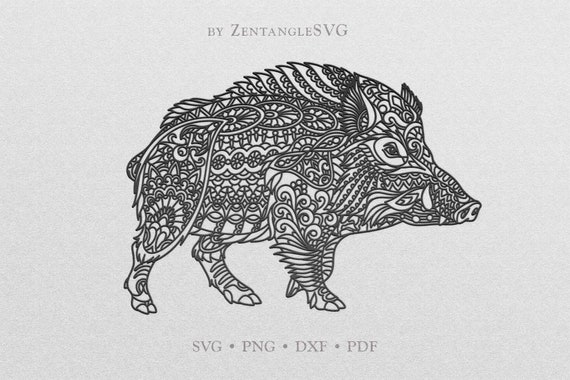The image features a detailed pen or pencil drawing of a pig set against a white background. The pig is uniquely decorated with intricate black-and-white patterns, including swirls and circles, covering nearly every part of its body except for its teeth and nails. The pig appears to be in motion, walking towards the right. Above the animal, the text "by Zentangles SVG" is written in gray, with additional file format abbreviations "svg.png.dxf.pdf" placed beneath the pig. The combination of artistic detail and textual elements suggests a design that could be used for various digital applications.